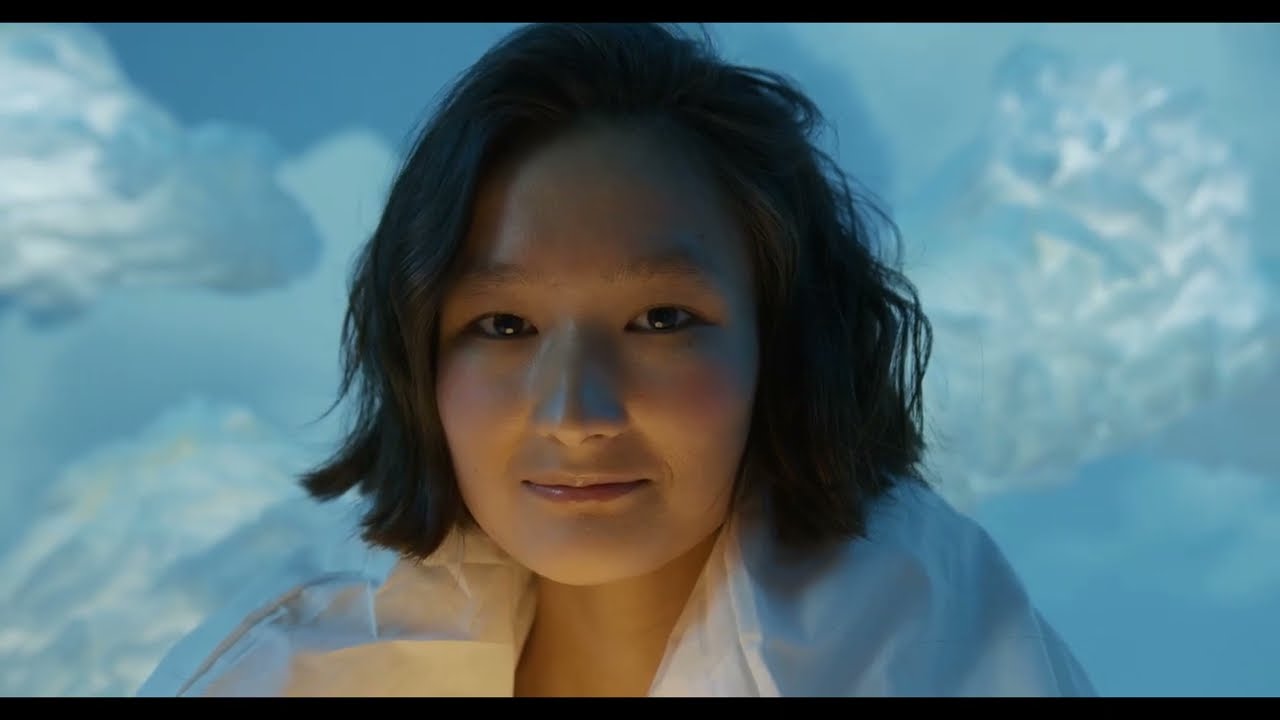The photograph captures a young woman of Asian descent with short, dark bobbed hair that grazes the bottom of her chin, parted at the side. Her complexion is tan, and her high cheekbones and straight nose are accentuated by her subtle, flesh-colored lips, which are pursed into a soft smile. Her monolid eyes, dark brown and inquisitive, gaze directly forward. She is adorned in a puffy, white jacket that envelops her shoulders and climbs up to her neck, adding to her winter-ready appearance. The background exudes an ethereal quality, with a light gradient of blue interlaced with billowy, white clouds that carry hints of dark gray. This luminous setting, which some might describe as evocative of an igloo or an ice cave, frames her with a sense of otherworldly calm and wonder, making the viewer almost feel the crisp, cold air surrounding her.